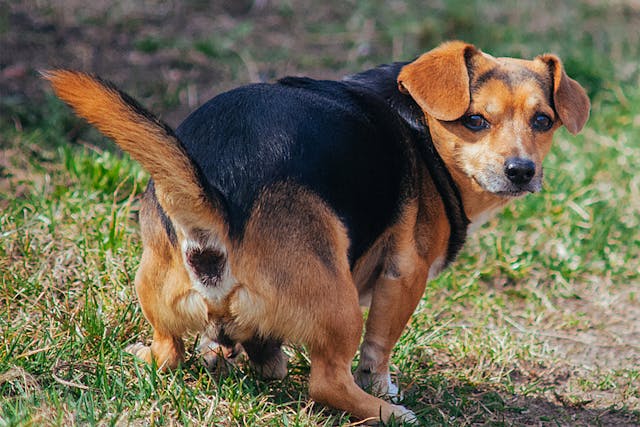A realistic, horizontal photograph taken outdoors during the day features a small brown and black dog, possibly a beagle and chihuahua mix, poised as if about to defecate on a grassy lawn. The grass, three to four inches tall, is mostly green with beige patches, appearing lighter in the front and darker towards the back. Positioned centrally, the dog has a black coat on its back and a reddish-brown hue on its face, legs, and rear. It is squatting with its tail raised, exposing its rear end and orifice, clearly about to relieve itself. The dog looks back over its right shoulder directly into the camera with its mouth shut, its expressive brown eyebrows adding to its alert, slightly unsettling gaze. The detailed depiction captures the dog's entire posture and setting vividly, creating a candid, if somewhat uncomfortable, moment frozen in time.